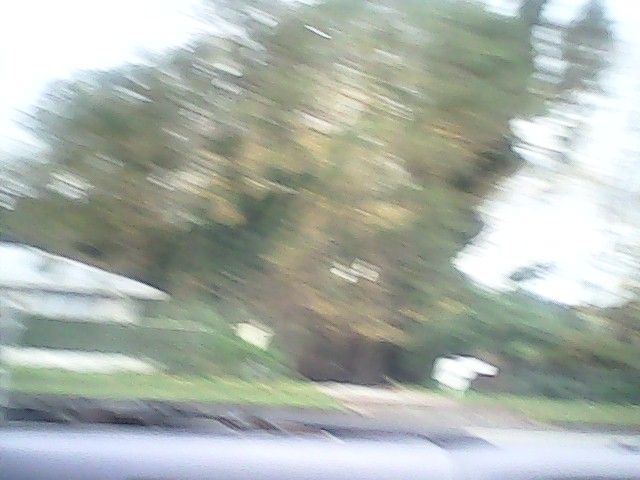The scene is an outdoor daytime capture taken from inside a moving vehicle through the windshield, displaying a highly blurred image. Central to the photograph is a group of trees, standing about three to four stories high, with leaves transitioning to yellow but mostly green. Toward the left of the center, a single-story white house with a white roof is seen in the background, nestled against a green, flat grassy lawn. On the right side, there are some white mailboxes next to a light tan concrete driveway that leads to the house. The sky, visible in the upper right corner, is overcast with fluffy white clouds. The foreground features the vehicle’s dash or window frame, and the dark gray asphalt street stretches from the lower left to the lower right across the image. The entire photograph is notably blurred and streaky, suggesting it was taken while the vehicle was in motion.